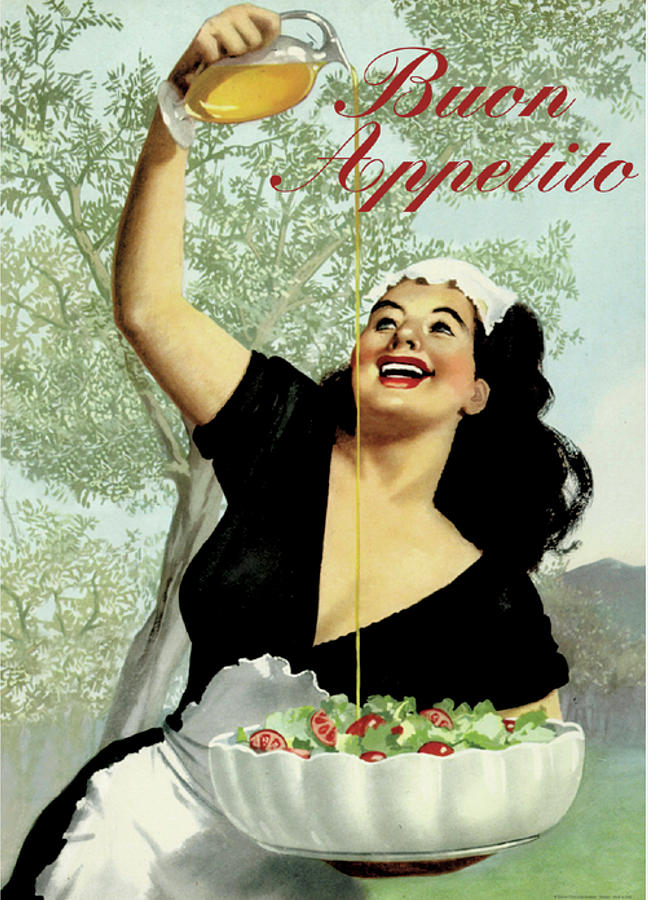This vintage-style illustration depicts a joyful woman outdoors, standing beneath a large tree with a blue sky overhead. She has dark, wavy hair, and wears a black dress with a V-neck and short sleeves. A white apron is tied around her waist, and a handkerchief sits atop her head. The woman, with a radiant smile accentuated by her bright red lipstick, is portrayed looking up as she pours golden olive oil from a glass decanter into a large, wide, and white salad bowl. The salad is vibrant with green lettuce and red tomatoes, visibly catching the dripping oil. The image evokes an old-school Italian home kitchen feel, and the text "Buon Appetito" is prominently displayed in red script at the top right corner.